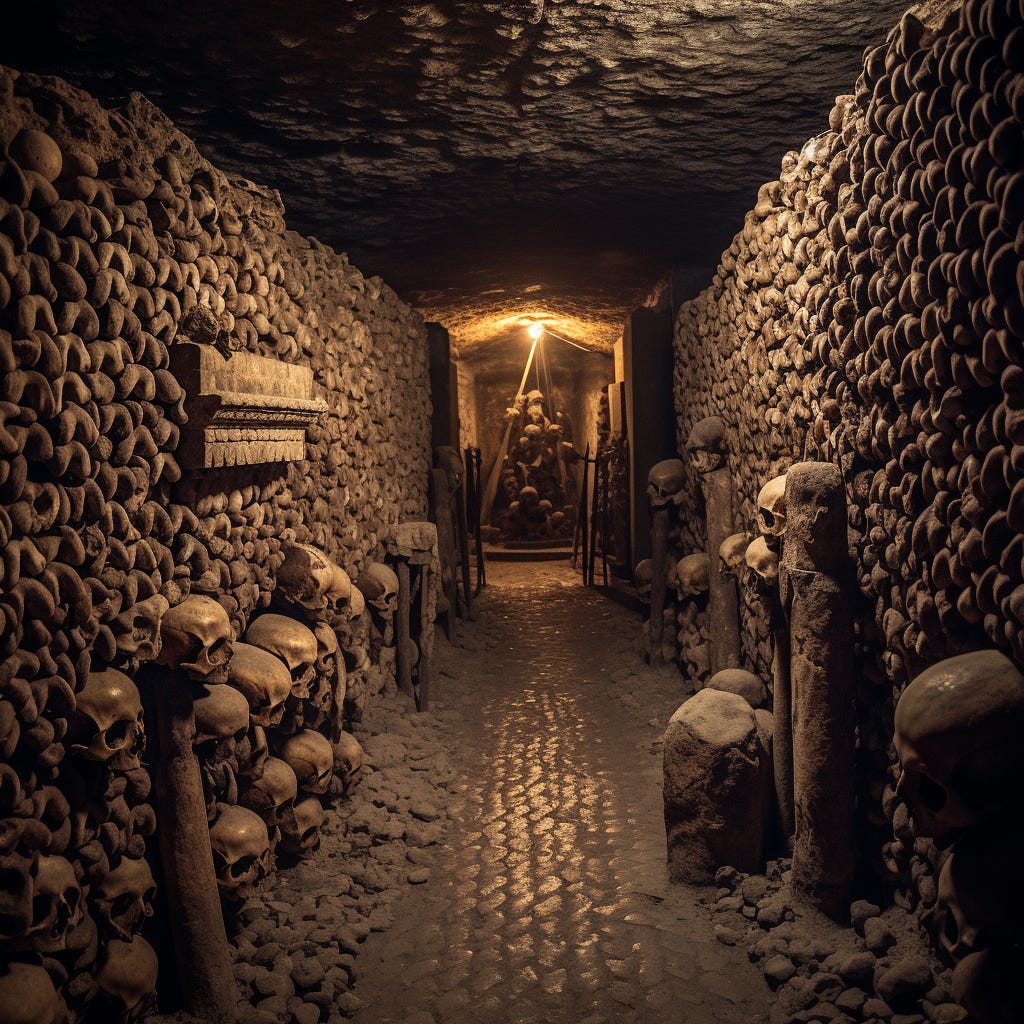The image depicts a dark, narrow tunnel resembling a dungeon or an ancient historical site. The ground is covered in gray and black dirt and stone, creating a dingy, unwelcoming atmosphere. The tunnel is flanked by walls made of gray and black stone, which have a texture reminiscent of small mounds or cushions. Human skulls are a prominent feature in the image, with many stacked to the left of the pathway and others mounted on pillars or embedded into the walls. Far in the background, lit by a ceiling light, stands a statue of a wizard holding a large staff, adding a hint of mysticism to the eerie setting. The tunnel leads to a stone doorway, beyond which more skulls can be seen, enhancing the macabre and historical feel of the scene.